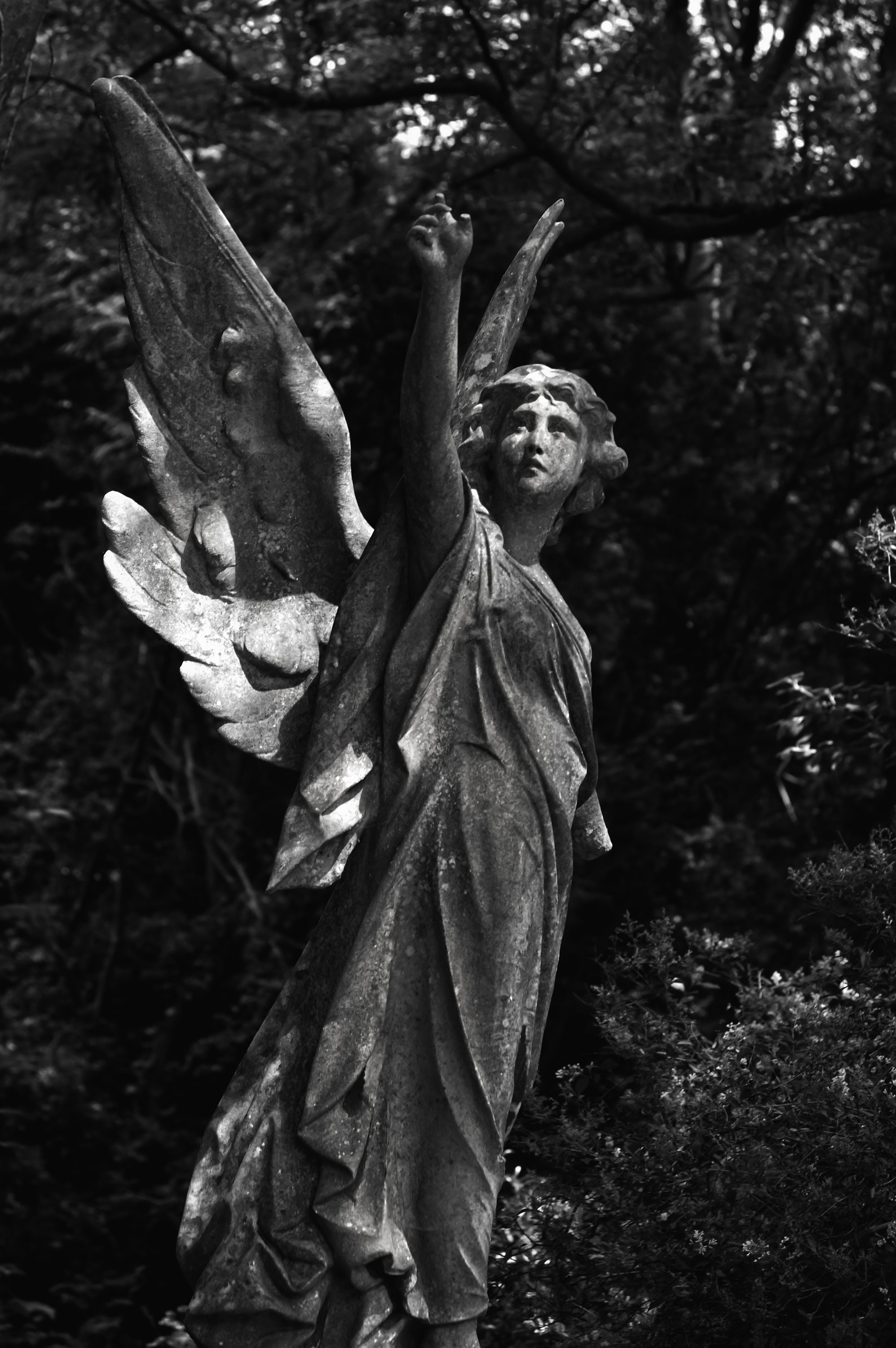In this meticulously detailed black-and-white photograph, an impressive stone statue of a female angel commands the center of the image, slightly to the left. The angel, adorned in a toga-like gown with flailing layers that may have originally been white, exudes an ethereal presence amidst a densely packed outdoor background of trees and bushes. This intricate statue features large, pointed wings spread apart, with the upper halves more prominently visible. Illuminated subtly as if by daylight, though the sky remains indistinguishable due to the monochromatic scheme, the angel gazes and points upward with her right hand. Notably, the statue's index finger and thumb have been broken off. Her hair is styled in wavy, chin-length curls, adding to the lifelike quality of the carving. The overall clarity of the photograph, which has a distinctly modern feel, accentuates the details of the angel's serene face and the elaborate foliage behind her.